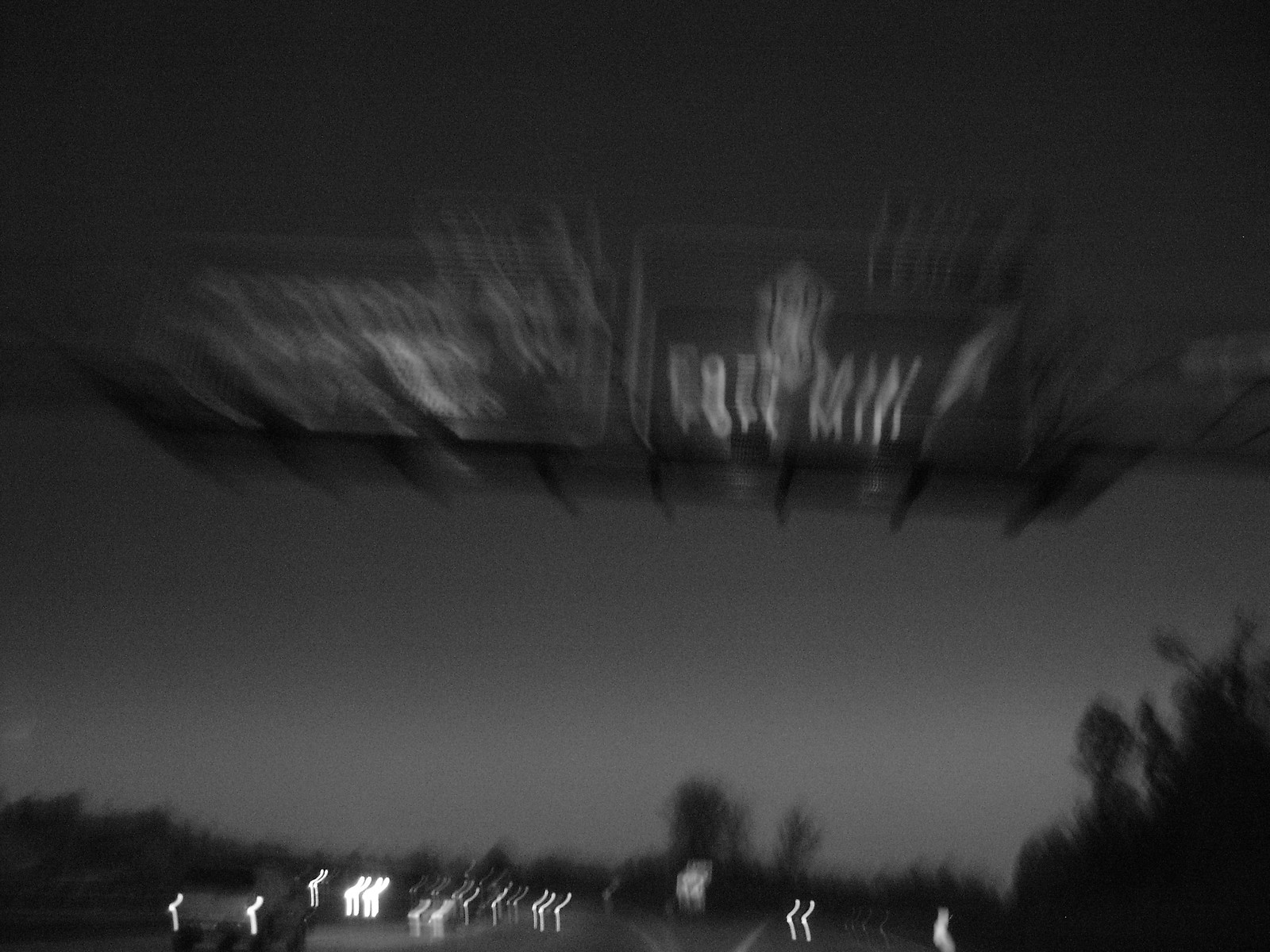This is a very blurry black-and-white photograph, likely taken at night or dusk from a moving vehicle. The image captures two major roadways with an overpass above, featuring two indistinct, blurred signs — one of which seems to indicate an exit. The overall scene is out of focus, creating an impression of motion and slight duplication of elements. Headlights and taillights of several cars streak across the image, with one visible truck with a canopy heading in the opposite direction. Trees frame the image, mostly to the right, extending to black at the skyline. The sky transitions from light gray near the horizon to dark gray above, possibly obscuring a roof with unreadable text. The overall moody atmosphere feels reminiscent of a surveillance camera capturing the frenetic life of a nighttime freeway.